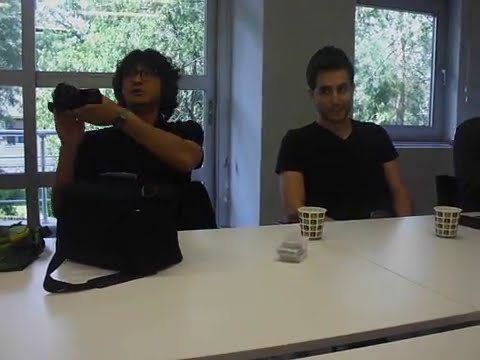This square photograph captures an indoor scene of two young men sitting at a long, white office table. Positioned in front of several large square windows that reveal a bright, sunny day with trees outside, the setting suggests a conference or meeting room. Both men are dressed in black short-sleeved t-shirts. 

The man on the left, who appears to be of Asian descent, has slightly curly, shoulder-length black hair and wears glasses. He is looking up and to the left, with his hands raised and holding a black object, possibly a video camera, which he seems to have taken out of a nearby black bag with a strap. A watch is visible on his wrist.

To his right sits a man with short black hair, fair skin, and possibly of European or Middle Eastern descent, also wearing a black t-shirt. He is similarly focused in the same direction as his companion, gazing intently upwards. On the table in front of them are two white paper cups adorned with square designs. The photo conveys a sense of anticipation or preparedness, as if they are about to begin a presentation or record an event.